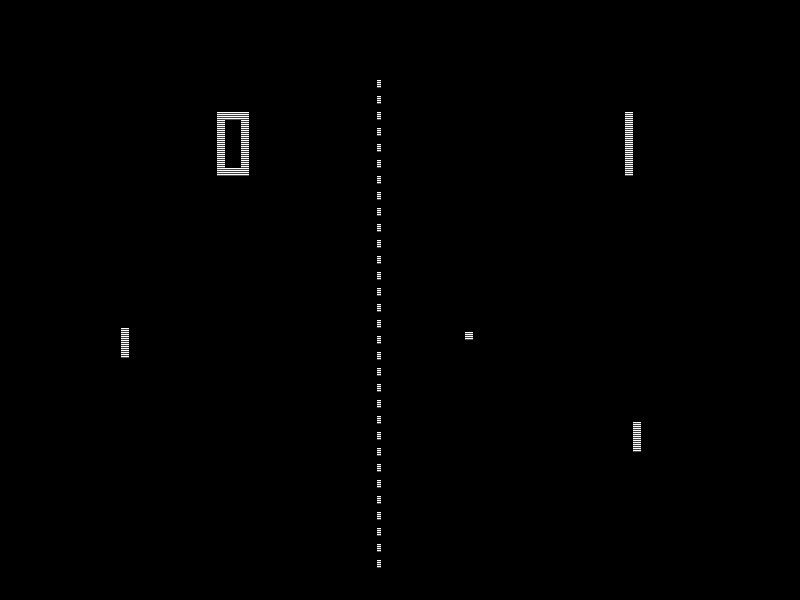The image is a screenshot of the classic video game Pong, developed by Atari in the early 1970s. The screen features a stark black background typical of the 8-bit era, focusing on minimalist visuals. At the center, a dashed vertical line represents the "net," extending slightly below the midpoint but prominently dividing the screen. 

On the left-hand side, a rectangular paddle is positioned near the middle, while on the right, a slightly unequal paddle is situated closer to the bottom. The paddles are poised for action, awaiting the game's iconic "ball," a small dot currently moving leftward from the right side of the screen. Above the net, the score is displayed: a "zero" on the left and a "one" on the right, indicating the progress of the game. The simplicity and crispness of the image capture the essence of Pong, symbolizing the rudimentary yet revolutionary beginnings of video gaming.